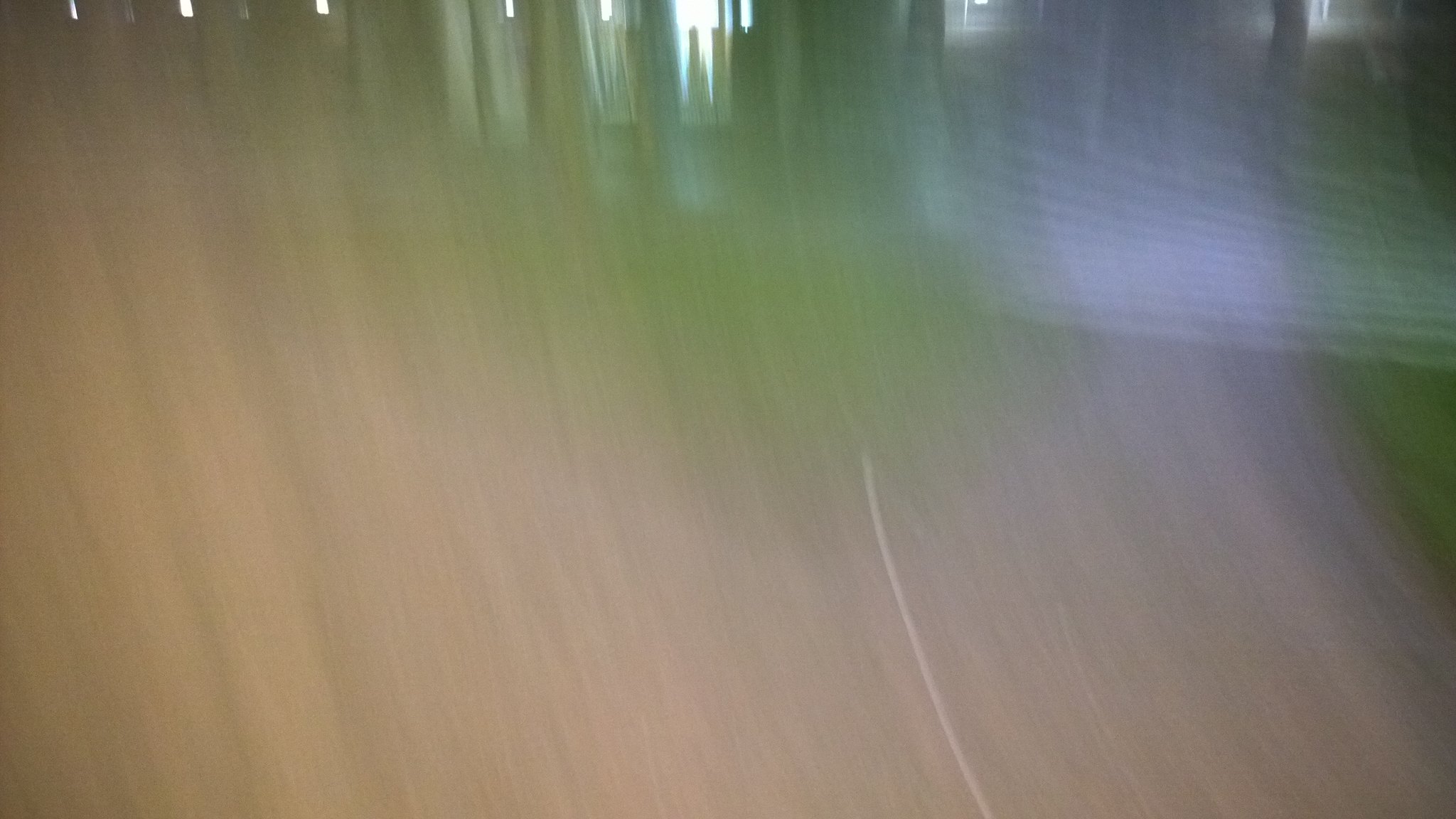This image captures an abstract, unintentional photograph taken with movement, resulting in a fully blurred scene. The distorted streaks of brown indicate a wooden floor, giving the impression of a hurried motion across the room. Central and slightly to the right, a whiter, vertical blur extends from the bottom to the top, possibly indicating a wall or another vertical structure. Towards the top of the image, several brighter, rectangular shapes create the faint suggestion of windows, their contours completely obscured. Above these shapes, at the very top edge of the photo, is a series of bright rectangles, adding to the overall abstract composition of the image.